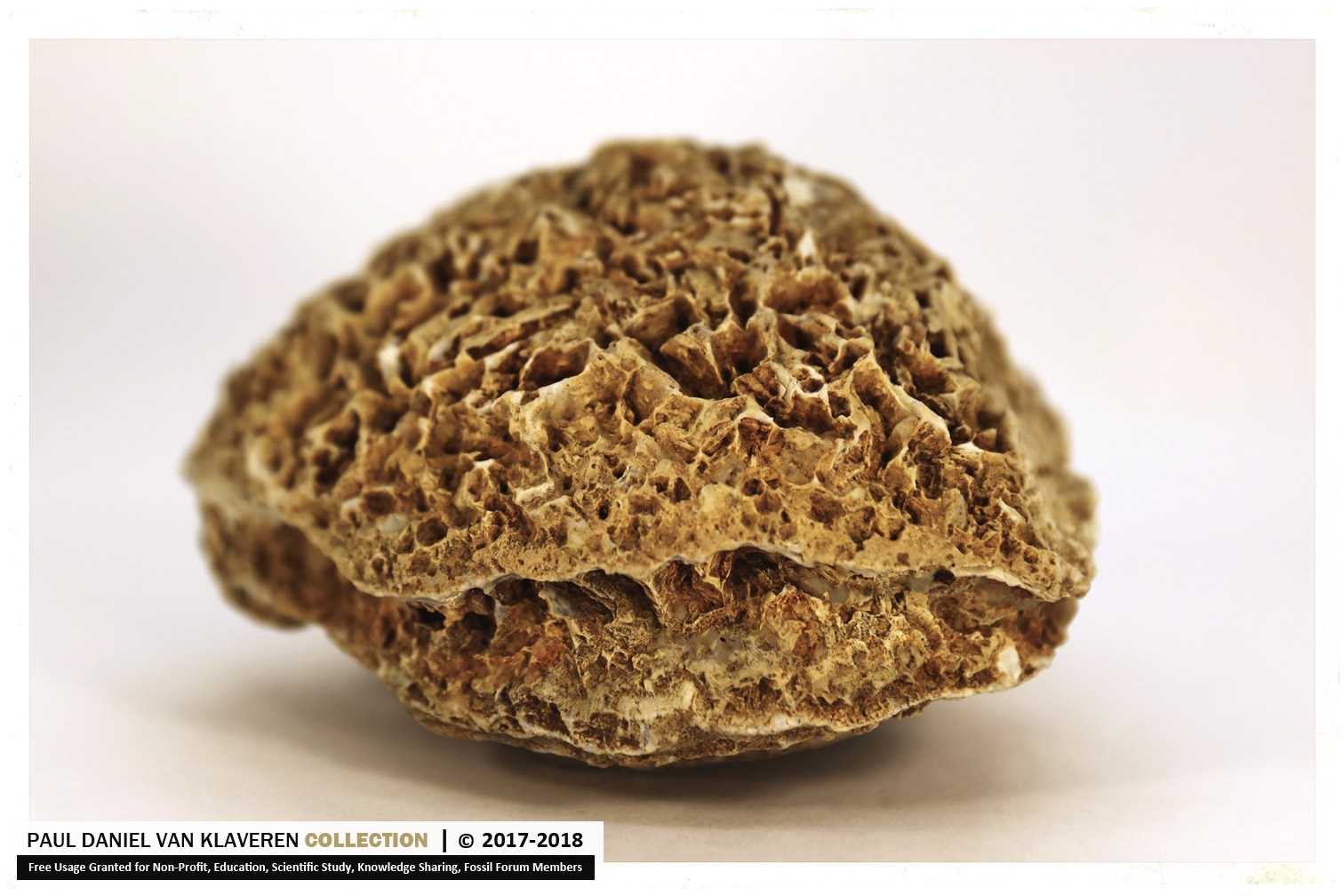In the center of this rectangular image, measuring approximately five inches wide by three inches high, stands a highly detailed, porous, and irregularly oblong object that resembles either a stone or a piece of coral. The object, roughly one to two inches tall and two to three inches wide, features a light brown color with diverse textural elements—ranging from darker brown grooves and deep gaps to lighter tan and white shades—giving it a truffle-like, cratered appearance. The background is a light off-white with a pinkish hue, and a shadow is cast below the object, adding depth to the image. In the lower left-hand corner, there's a white rectangular text box with black text reading "Paul Daniel Van Cleveren" followed by the word "Collection" in gold. To the right of this is a black vertical line and a black letter "C" inside a circle, indicating copyright, along with "2017-2018". Below this text, a black rectangle contains white text that states, "Free Usage Granted for Nonprofit Education, Scientific Study, Knowledge Sharing, Fossil Forum Members."